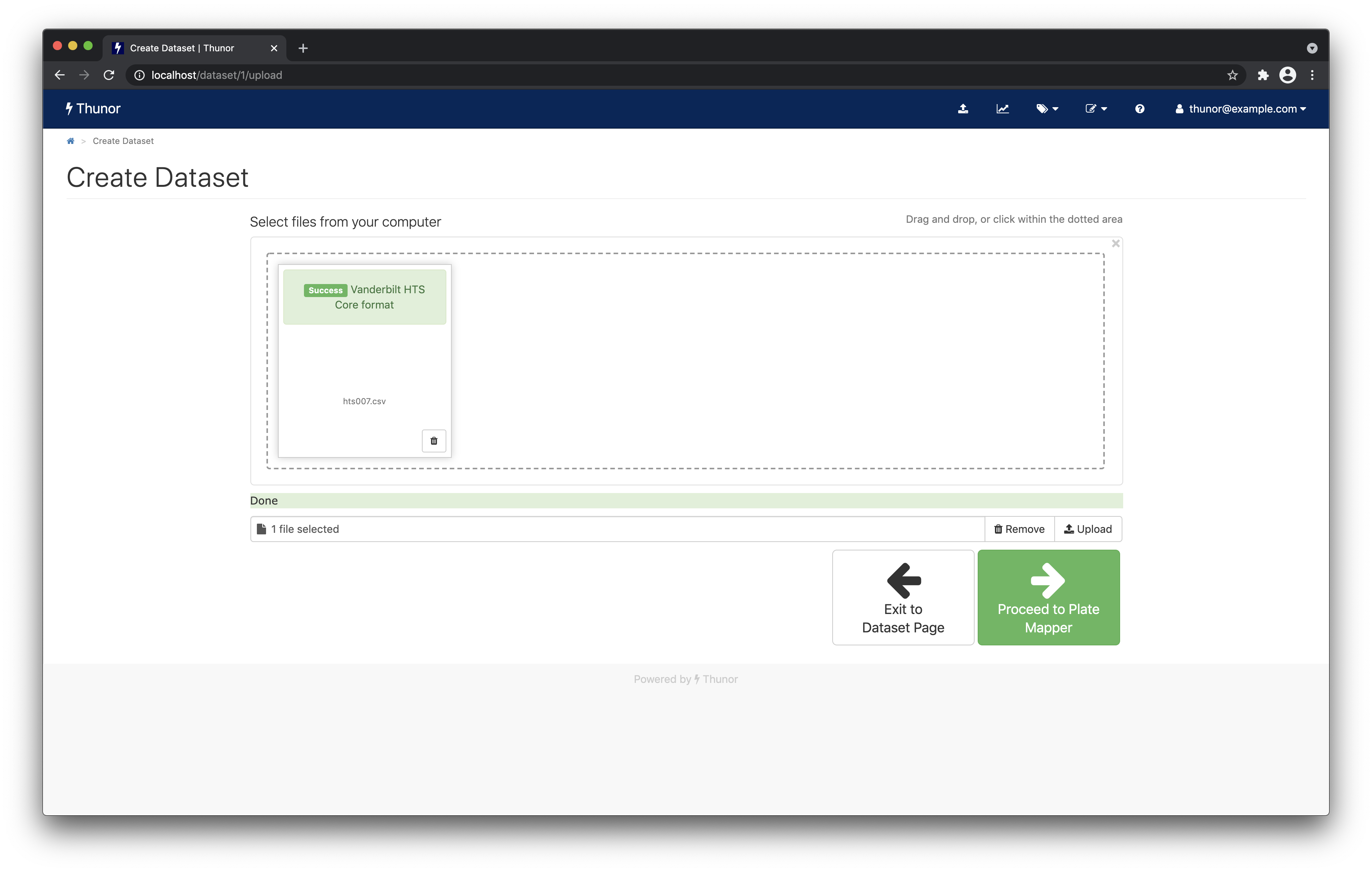**Screenshot of Thunor Data Editing Tool Interface**

This screenshot captures the interface of a data editing web tool named Thunor, showcased by its position in the browser tab where it reads "Create Dataset Thunor." The URL in the address bar indicates a local development environment, with "localhost/dataset1/upload" clearly visible.

In the top-left corner of the screen, there are three horizontally arranged circular icons reminiscent of a traffic light, colored red, yellow, and green, characteristic of Mac OS window controls. Immediately below these, a prominent label reads "Create Dataset."

Central to the interface is a rectangular file upload section, highlighted by a green banner with the message "Success." This indicates that a file named "HTS007.csv" has been successfully uploaded. The green banner references the specific format required, denoted as "Vanderbilt HTS core format."

Within the rectangular section, text instructs the user to "select files from your computer." Below, a confirmation states "1 file selected," accompanied by a "remove" button for managing the uploaded file.